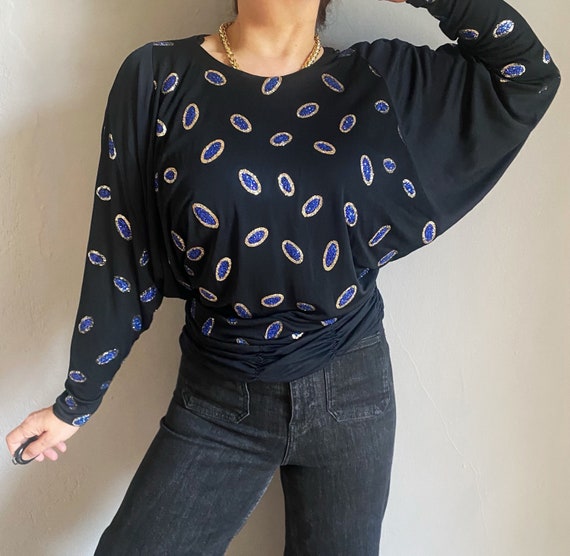The image captures a female model from the neck down to her knees, set against a white background shaded with hues of gray. She is showcasing a distinctive, long-sleeved black shirt that is notably baggy under the arms. The shirt features unique blue oval patterns, each bordered with a very light yellow, scattered across the fabric. Accompanying the shirt, she wears dark, faded black jeans equipped with front pockets. Around her neck, there is an elegant gold necklace, adding to the stylish ensemble. The model, who has light-colored skin and visible wisps of dark hair, has her left arm raised, concealing her hand, while her right arm is down, holding an instrument of some sort between her thumb and index finger.